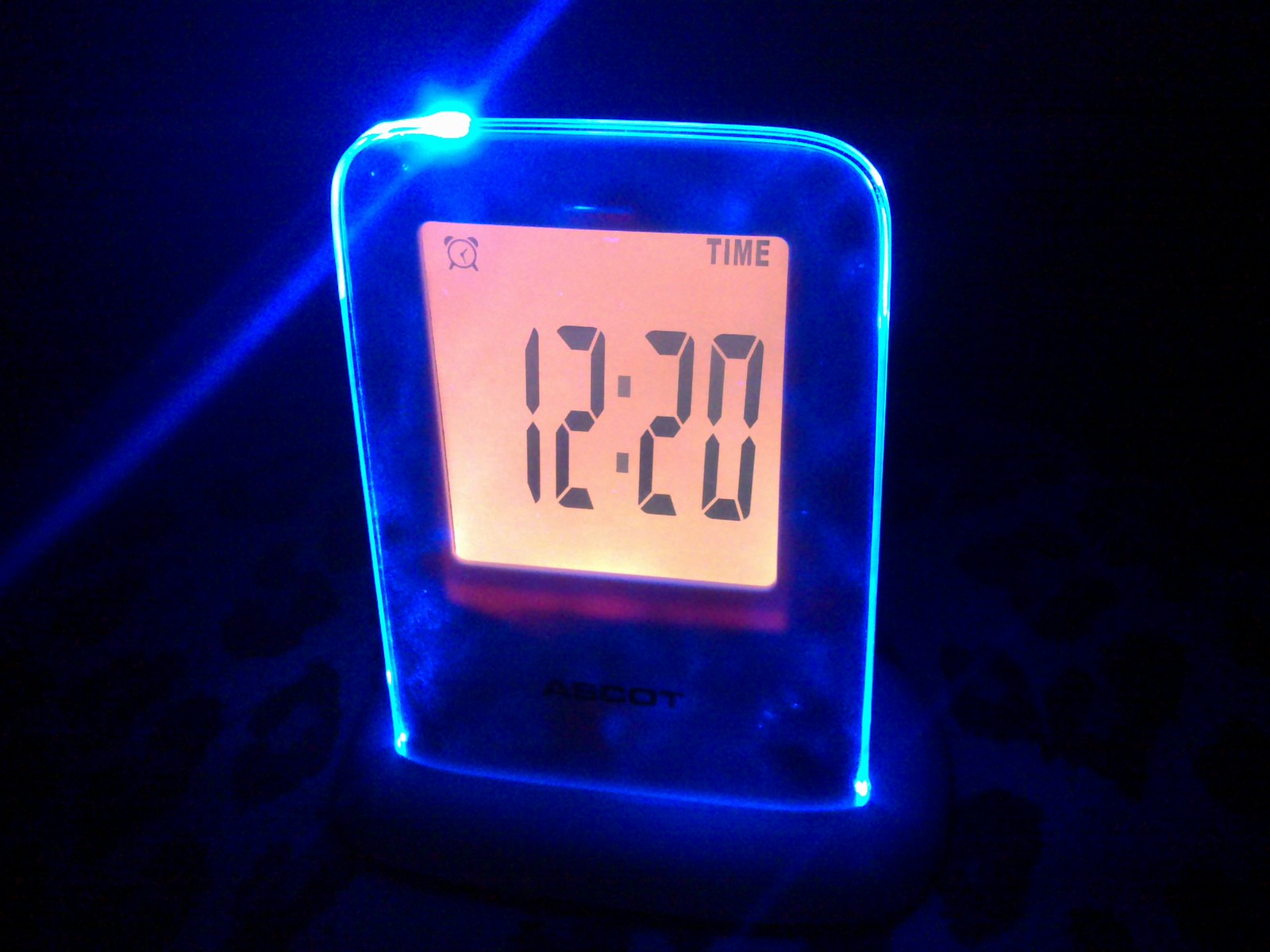A digital clock is prominently displayed in the center of the image, casting an orange glow from its illuminated face. The time reads 12:20, with a small alarm clock icon situated in the top left corner of the display, while the word "TIME" is displayed in the top right. Surrounding the central display, the clock's body appears to be made of a semi-transparent black material, suggesting it could be plastic or glass. This dark, reflective surface is contrasted by a subtle, glow-in-the-dark illumination that borders the clock face, creating a distinctive halo effect in the otherwise dark environment. A small blue light can be seen in the top left area, adding a cool contrast to the warm orange display. At the bottom of the clock's face, the brand name "Ascot" is visible. Below the clock, a pattern resembling cheetah print can be discerned, though its exact nature is unclear.